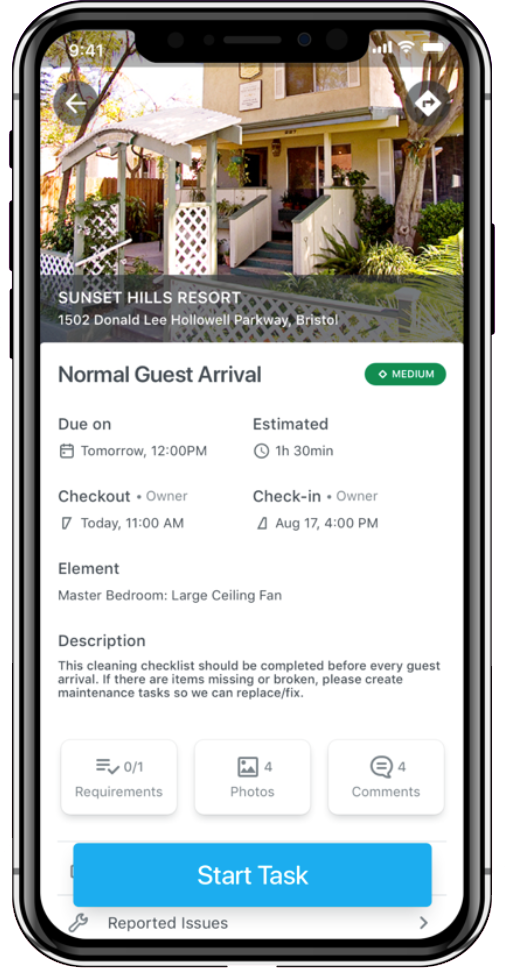**Detailed Caption:**

The image showcases a smartphone screen, zoomed in to reveal its contents. The phone, possibly an older model iPhone with a silver bezel, displays an itinerary for an arrival at the Sun Hills Resort. The resort's image is prominently featured, presenting a pristine, whitish-yellow building with a small canopy, a welcoming walkway, and lush trees, evoking a serene atmosphere. The detailed location of the resort is listed as 1502 Donnelly Hollowell Parkway, Bristol.

Further down the screen, an entry labeled "Normal Guest Arrival" is highlighted, showing a green status indicator suggesting the task is due tomorrow at 12 p.m., with an expected duration of an hour and 30 minutes. The checkout was scheduled for today at 11 a.m., while the check-in occurred on August 17th at 4 p.m. The element noted is the "master bedroom, large ceiling fan."

A descriptive section emphasizes the importance of completing a cleaning checklist before each guest's arrival, with instructions to report any missing or broken items so maintenance tasks can be initiated. The interface also includes three sections: "Requirements" (0 of 1 completed), "Photos" (4 uploaded), and "Comments" (4 entries). At the bottom, an option to "Start the Task" is visible, suggesting the checklist is part of a task manager, likely used by resort staff or maintenance workers.

The background of the smartphone screen is predominantly white, ensuring the details and images stand out clearly for easy reading and navigation.